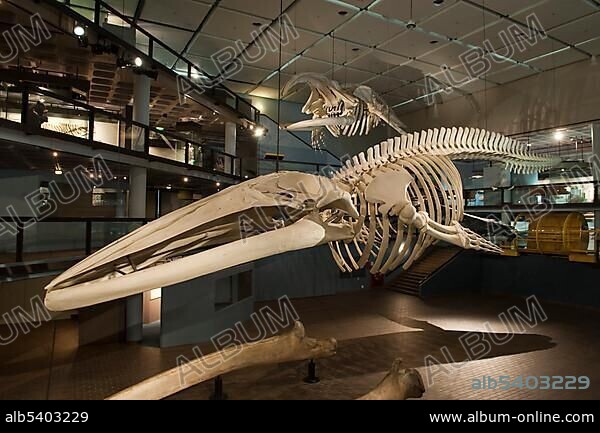The photo depicts the interior of a modern museum featuring dinosaur exhibits. Dominating the foreground is a large dinosaur-like bird skeleton with an enormous head and beak extending almost half the width of the image. The bird's actual body is relatively small, with about 15 ribs in its rib cage, representing only about a third of the length of the head. Extending above the rib cage is a long spine forming a tail roughly the same length as the beak. Suspended from the ceiling with ropes, similar skeletons are visible in the background, suggestive of aquatic dinosaurs with front flippers instead of legs. The viewing area includes two stories with black railings and curved ceilings finished in gray and white tiles. The sleek, modern design of the space adds to the atmosphere of the museum. The image is watermarked with the text "album" and marked with "ALB 5403229" in the bottom left corner and "www.album-online.com" in the bottom right, indicating it is a stock photo from album-online.com.